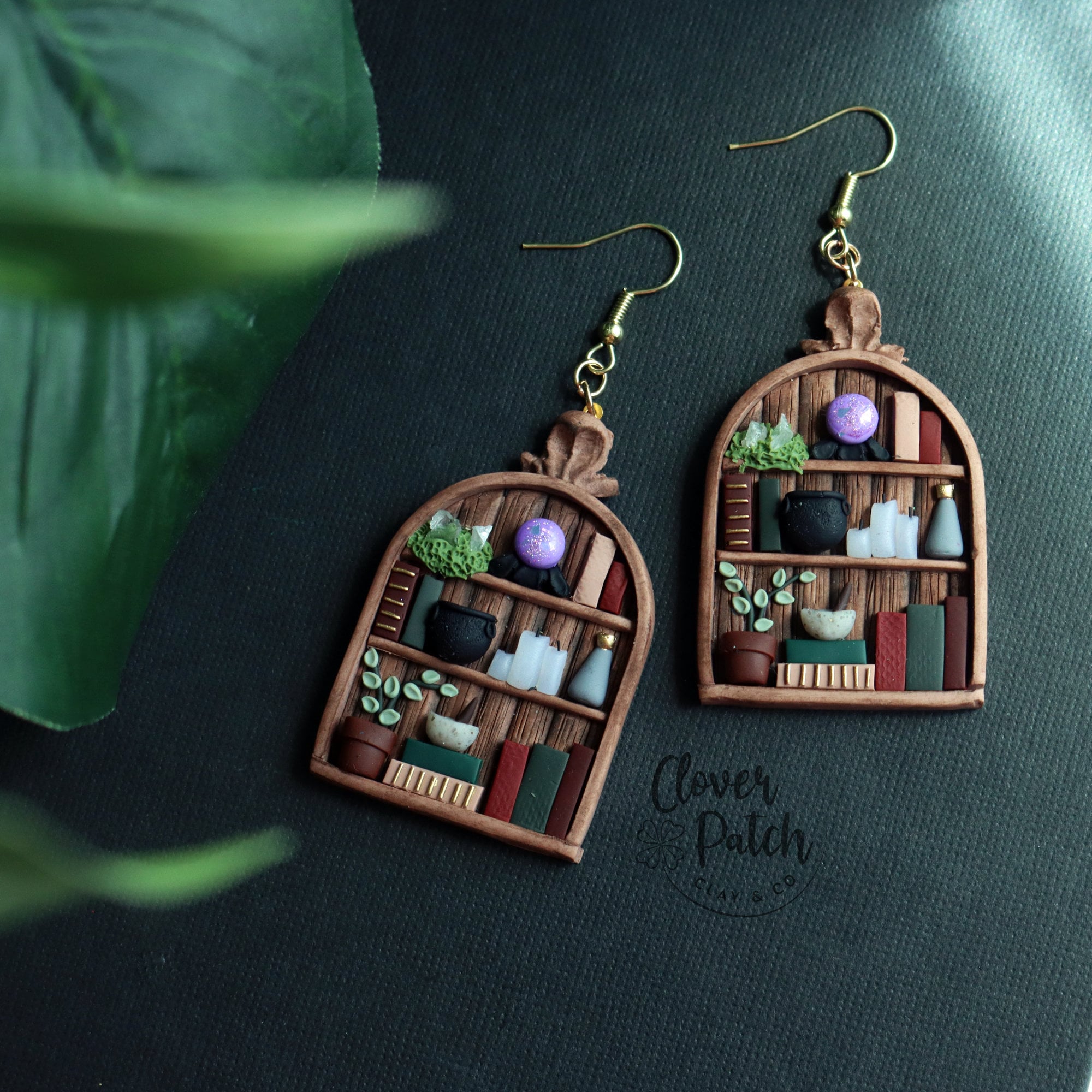This image showcases a pair of unique, handcrafted earrings designed for pierced ears. The earrings, featuring gold shepherd's hook wires, are intricately fashioned to resemble miniature bookshelves, each with three tiers. The top shelf on each earring includes a tiny potted plant with trailing leaves, a crystal ball on a black holder, and several books. The second shelf contains two books, a black bowl, three candles of varying heights, and a vase. The bottom shelf displays a potted plant with small green leaves, a small bowl atop two books, and three vertically standing books in green, red, and brown. Each earring's bottom tier also includes a black kettle and a mortar and pestle, items often associated with witchcraft. The background features a bluish-gray quilted fabric, upon which is written "Clover Patch" with a shamrock logo. Additionally, there are some artificial green leaves to the left of the earrings.